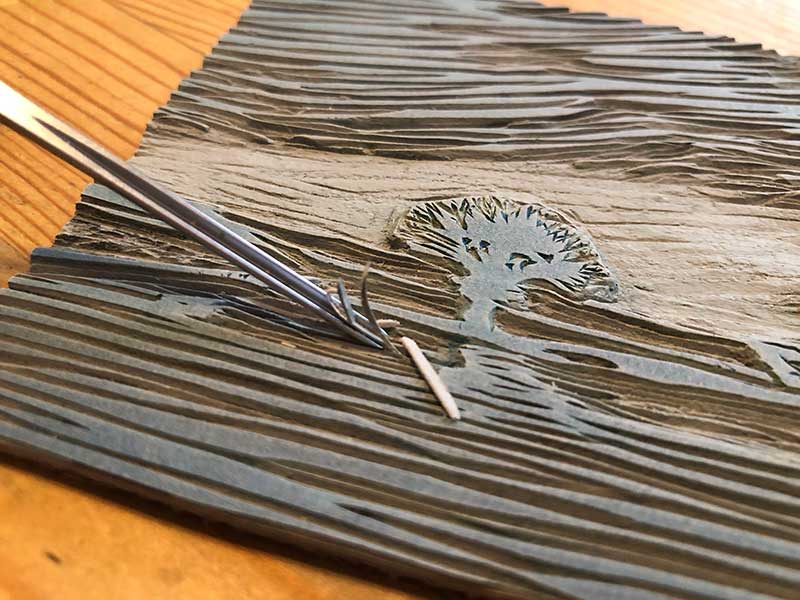The image depicts a partially finished wood carving scene on an orange wooden table. The central focus is a symbol of a tree that appears to be intricately carved out of a light brown piece of wood. The background of the carved wood resembles bark, adding to the natural, earthy aesthetic. Surrounding the tree, the wood shows signs of splintering and rough texture, indicating recent carving activity. Slightly to the right of the center, the carved tree stands out amidst the less detailed background.

On the left side of the image, there is a metal tool, possibly resembling very thin tongs or a small two-tine fork. The tool is positioned diagonally, resting on the wood, and appears to be actively carving, pushing up tiny pieces of wood and creating precise lines within the material. The overall scene has a minimalistic color palette dominated by browns and oranges, with a sense of artisanal craftsmanship in progress. Lines and cut marks are visible throughout the wood, suggesting the careful effort put into this artistic woodworking project.